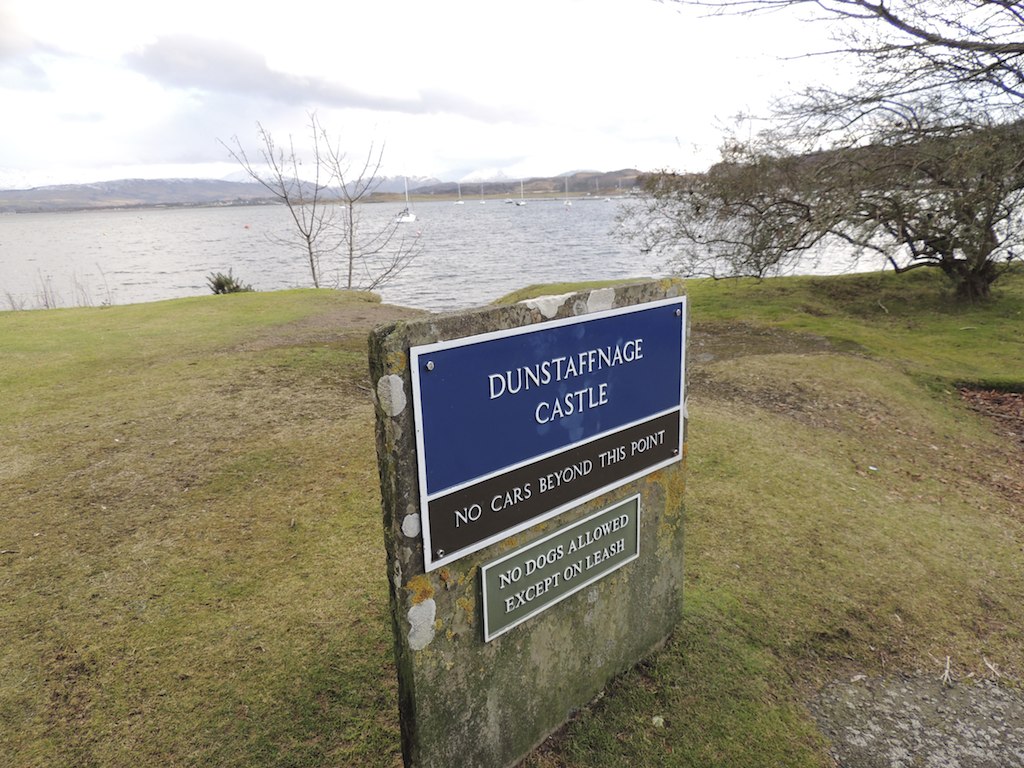This color photograph captures a serene lakeside scene dominated by a prominently placed sign in the foreground. The sign, mounted on a thin piece of stone, is composed of three sections: a blue top section that reads "Dun Staffnage Castle," followed by a black section stating "No cars beyond this point," and a green section indicating "No dogs allowed except on leash." The sign stands amidst a grassy area leading to the lake, where several white sailboats are anchored, their sails not hoisted. The lake's still waters reflect the overcast sky, which is slightly gray with larger puffy clouds, conveying a sense of calm. To the right of the scene, a small, flat-shaped tree adds a natural element, while in the background, low mountains rise gently, adding depth to the landscape. This picturesque setting beautifully combines natural and man-made elements, with a historic castle sign as the focal point.